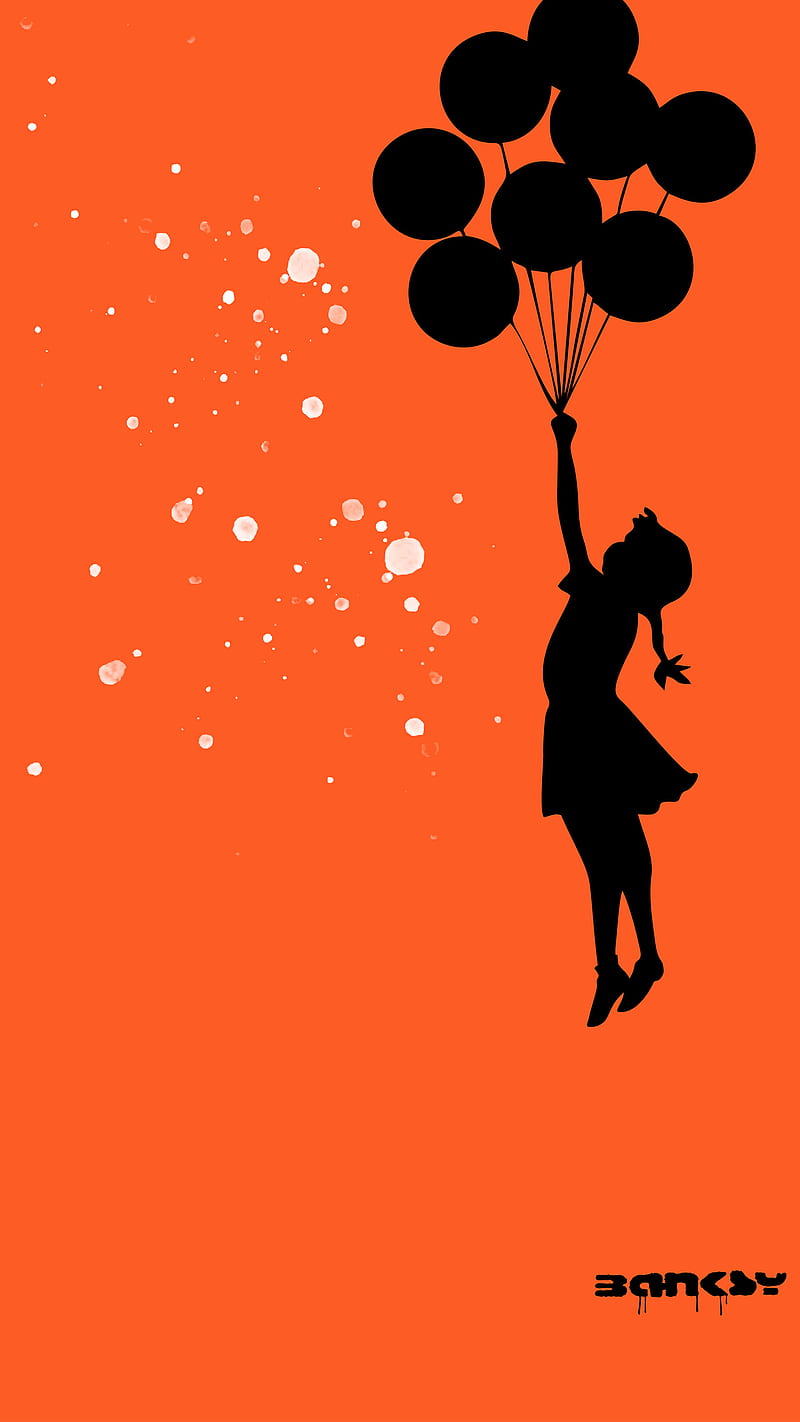In this captivating image, a vivid, bright orange background sets a vibrant scene, accentuated by splatters of white paint that evoke a sense of magic and whimsy. The central figure is a striking black silhouette of a young girl, reminiscent of Mary Poppins, with a ponytail or braid and a dress with shoes. She is lifted gracefully into the sky by eight helium balloons, all depicted in silhouette. Positioned just below the girl, a somewhat obscured inscription hints at the name "Yeon Kae" or possibly another name, with some of the letters appearing to drip like spray paint, adding an artistic and fantastical touch to this enchanting visual narrative.